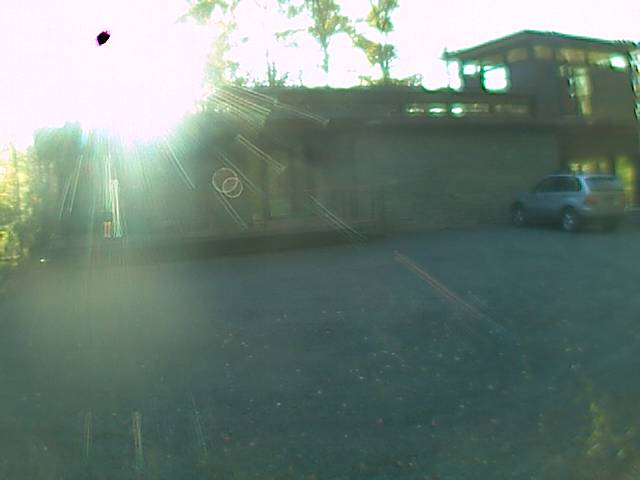This is an overexposed photograph of a building, possibly a home or a commercial structure, such as a ranger's office in a forest. The sun is shining through the trees in the background, casting an intense glare that dominates the image, particularly affecting the upper left side, which is almost impossible to view due to the brightness. This glare has caused artifacts, including circular light spots, and has even burnt the photograph, leaving a black spot where the sun is. The overall quality of the image is low, suggesting it may have been taken from a distance or as a screenshot from a webcam.

The building itself appears to be made of brown brick with numerous windows. There is a distinctive section with an extended roof that has windows lining it, and attached to it is a taller, squarish tower-like structure, possibly two floors tall, with many glass windows. This tower might have stairs leading up to a higher viewpoint, perhaps to overlook the surrounding forest. A single grey SUV is parked in front of the building, which sits on a large, paved asphalt driveway marked with standard lines. The doors of the building have windows displaying a green or yellow light. The photograph's blurriness and small size make it challenging to discern finer details.